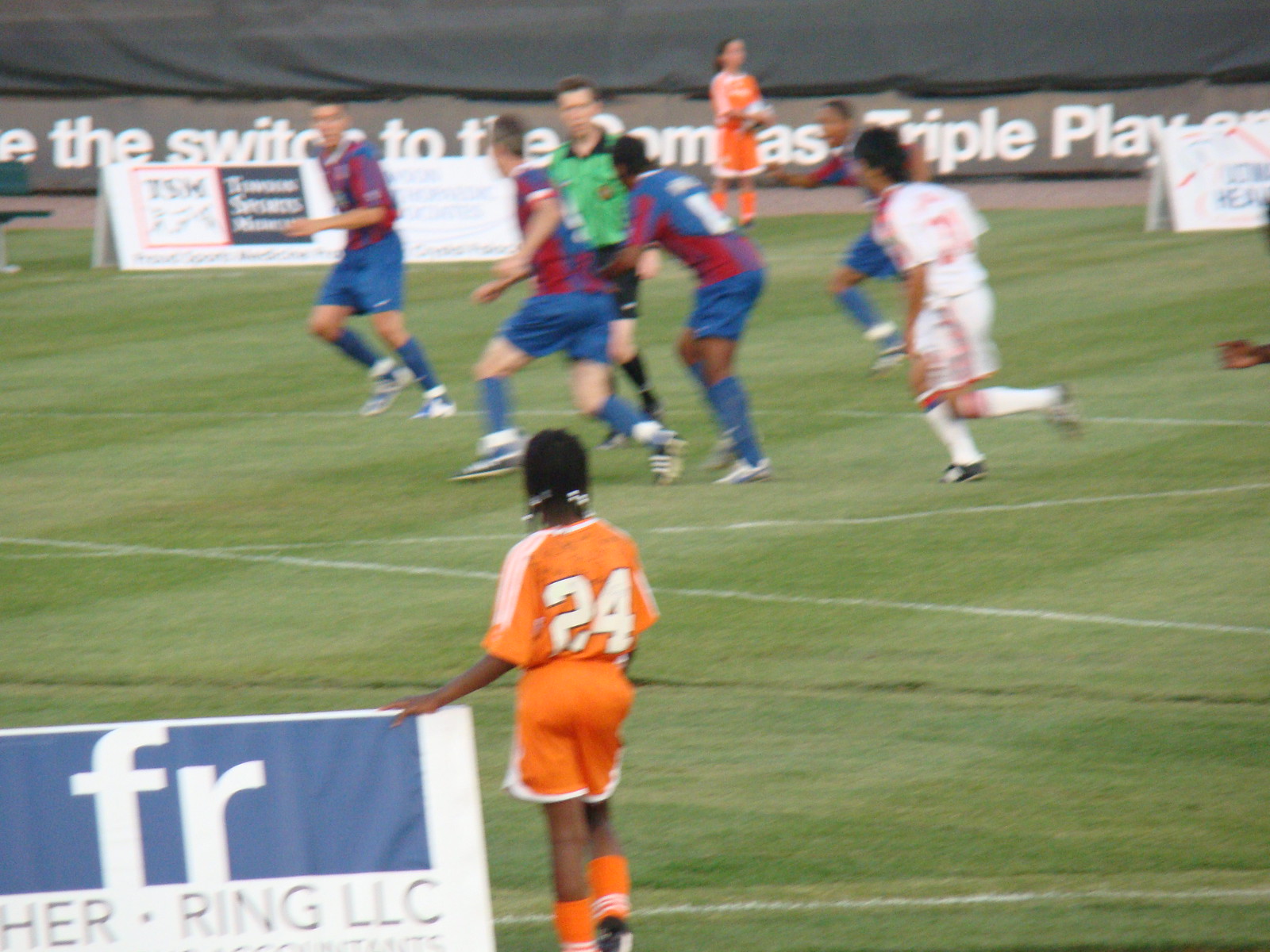This slightly blurry and out-of-focus action shot captures a lively soccer game being played on a large, grassy outdoor field. Central to the image are several men actively running, their movements creating a blur of energy and motion. They are divided into two teams, with one group donning blue and red jerseys and the other clad in white jerseys. A referee, distinguishable by his green and black jersey, is positioned in the middle of the action.

Flanking the field, spectators and possible substitutes are visible. Two females stand on the sides, their roles unclear, while a woman stands in the background by some signage, her arms crossed in attention. Additionally, a person dressed in an orange jersey with the number 24 on their back, sporting black cornrows, is seen near the signage, which includes the partial text "FR" in white font against a navy blue background.

The field itself features green grass with white painted stripes, and the edges are lined with signs and advertisements. The image, despite its blur, effectively conveys the dynamic and engaging atmosphere of a soccer match.